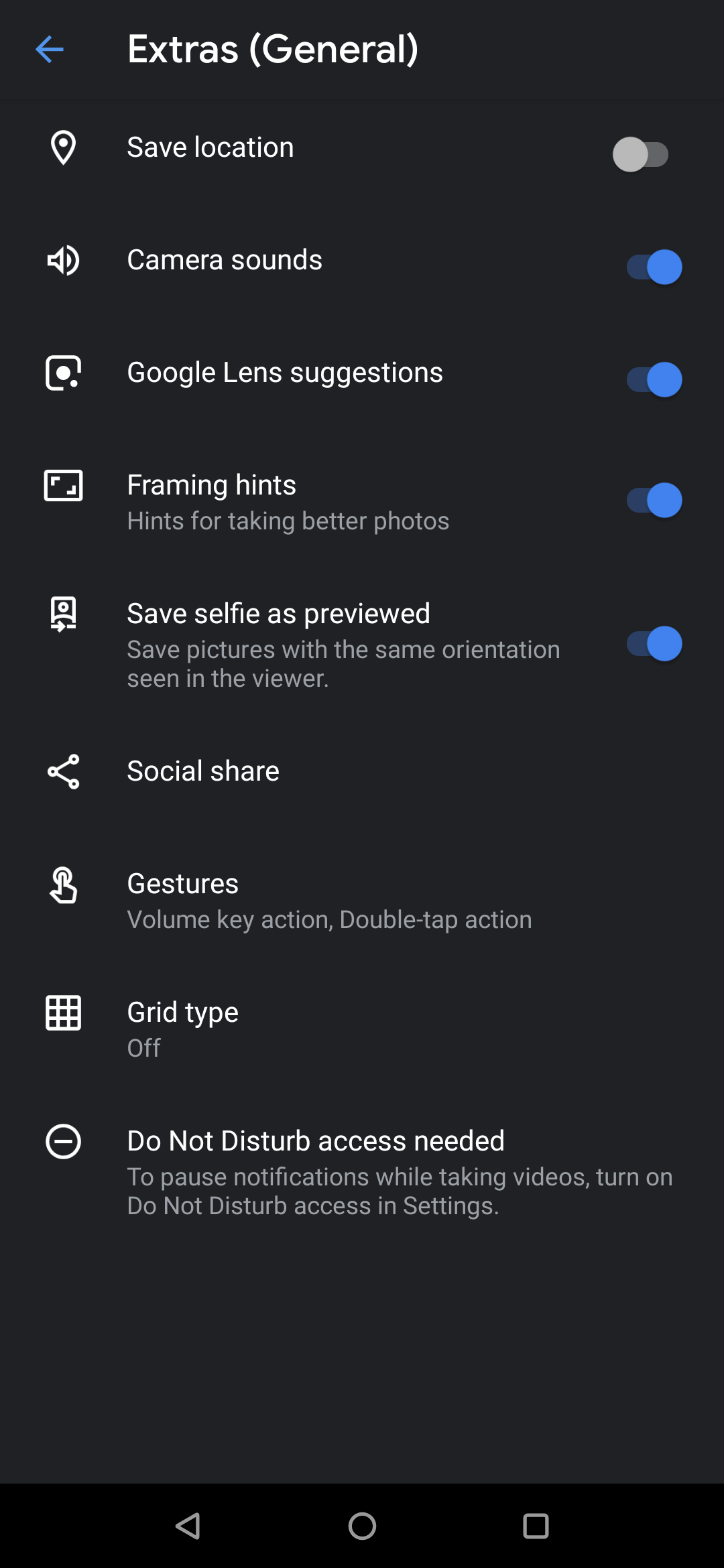This screenshot showcases a mobile application's "Extras (General)" settings page, featuring a sleek dark grey background complemented by a black footer at the bottom. 

In the upper-left corner, a blue arrow points to the left, adjacent to bolded white text that reads "Extras (General)". Below this header, a series of rows are presented with each row containing a white icon on the left, followed by white titles, and, in some cases, additional details in light grey text underneath the titles. 

1. **Save Location**: 
   - **Icon**: Map pin 
   - **Right Side**: A dark grey pill-shaped selection button with a light grey circle positioned on its left side.

2. **Camera Sounds**:
   - **Icon**: Volume symbol 
   - **Right Side**: A dark blue pill-shaped selection button with a bright blue circle on the right side, indicating it is activated.

3. **Google Lens Suggestions**: 
   - **Icon**: A white square with rounded corners, a missing bottom right corner, and two concentric circles in the center.
   - **Right Side**: A blue selection button.

4. **Framing Hints**: 
   - **Icon**: White rectangular shape with two white right-angle shapes in the top left and bottom right interior corners.
   - **Subtitle**: "Hints for taking better photos"
   - **Right Side**: A blue selection button.

5. **Save Selfie as Previewed**:
   - **Icon**: A selfie symbol
   - **Subtitle**: "Save pictures with the same orientation seen in the viewer"
   - **Right Side**: A blue selection button.

6. **Social Share**:
   - **Icon**: Share symbol
   - Additional rows with similar settings follow beneath this.

This arrangement provides a user-friendly interface for managing various settings related to photo-taking and sharing features within the mobile application.